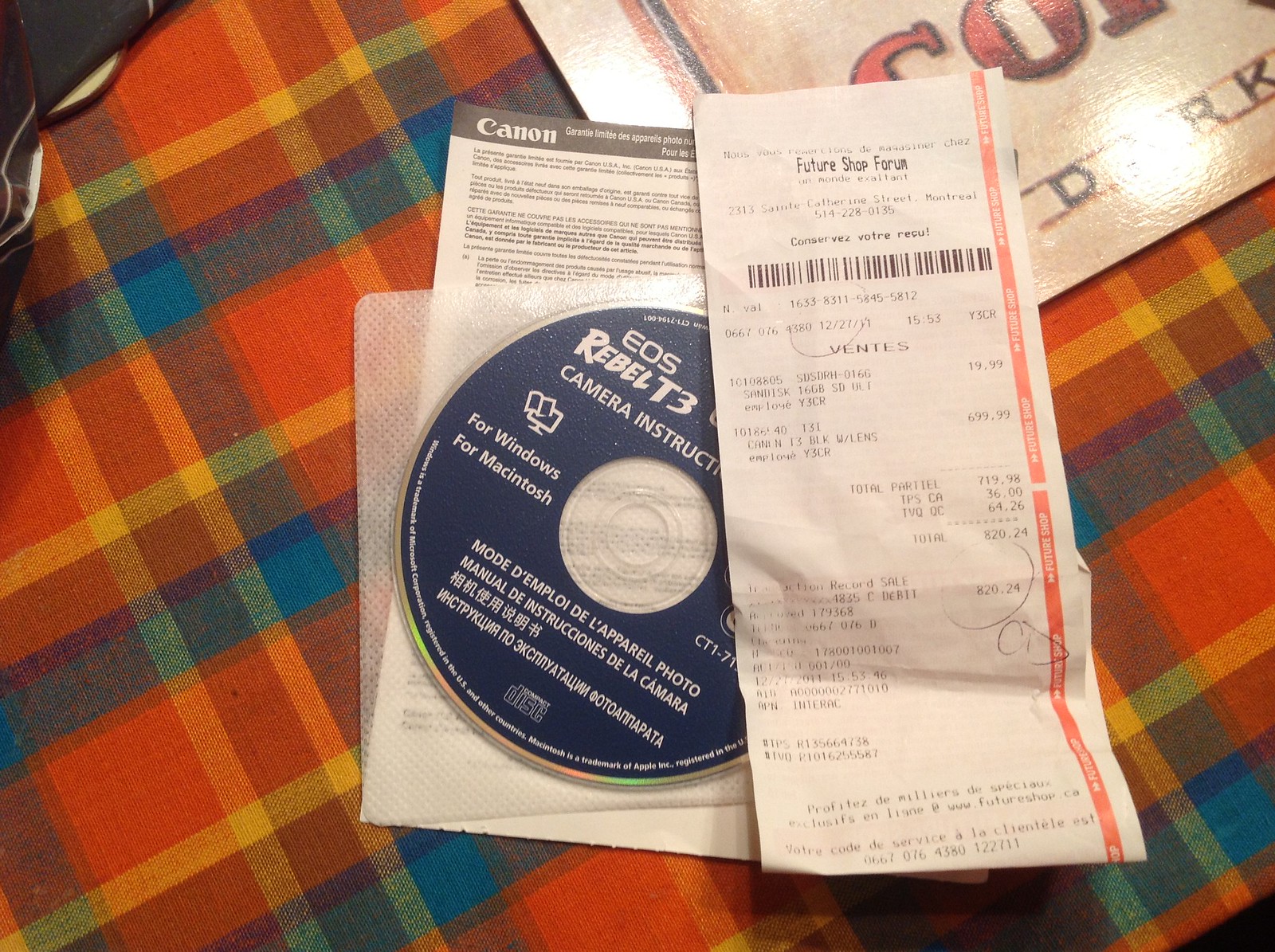This indoor photograph captures a detailed shot of a CD-ROM and a receipt, laid out on a flat surface. On the left side of the image, a CD-ROM is prominently featured. This CD-ROM is specifically for an EOS Canon Digital Rebel T3 camera and serves as an instruction manual for both Windows and Macintosh operating systems. The CD itself bears a navy blue label with informative text printed in a clear white font. It is securely placed inside a transparent sleeve, which rests on top of what appears to be the paper instruction manual for the same Digital Rebel T3 camera. A receipt is partially obscuring the right-hand side of the CD-ROM. The receipt, printed in French, indicates a purchase from FutureShop and originates from a location in Montreal.